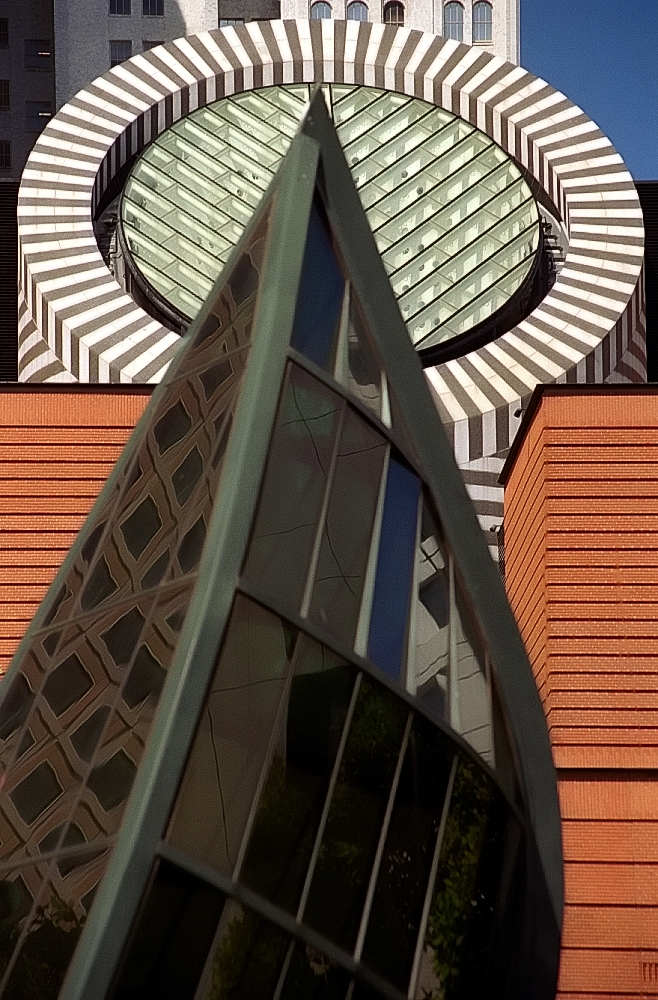The image showcases a striking example of contemporary architecture, featuring a combination of geometric shapes and contrasting colors. In the foreground stands a black metal building with glass accents, shaped somewhat like a bent triangular or teardrop form. Behind it, the scene becomes even more intriguing: a colossal circular structure dominates the background with bold white and gray stripes reminiscent of a zebra pattern. Within this circle, another smaller, glass-lined circle suggests a design akin to a sundial. Flanking these central structures are two red brick buildings, adding to the architectural diversity. Above it all, the top of a more traditional white building peeks through, possibly hinting at a city's skyline beyond. The fusion of all these elements creates a visually captivating and somewhat surreal urban landscape.